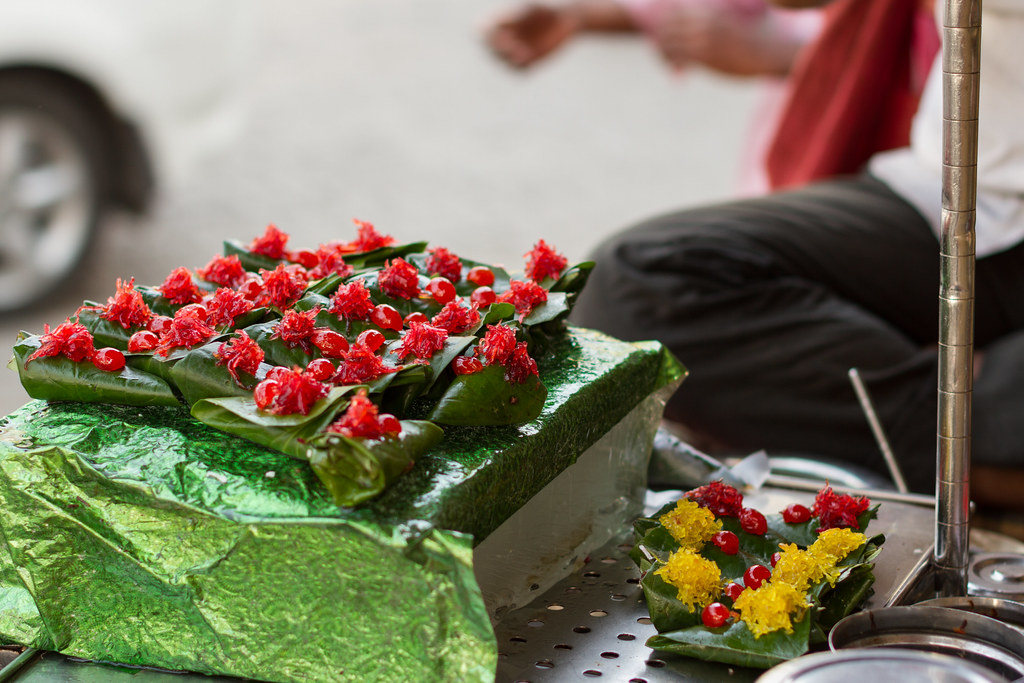The image shows a street vendor, partially visible with only their leg and shirt discernable, seated cross-legged and preparing an oriental dish. Central to the scene is a green box supporting a meticulously arranged display of green leaves, each meticulously wrapped around an unknown filling. These leafy bundles are topped with a cherry-red substance, possibly caviar or berries, adding a vivid contrast. Adjacent to the green box are pieces of the delicacy individually placed on a stainless steel grate with numerous holes. These pieces, similarly wrapped, are garnished with red and yellow elements, hinting at ingredients like tomatoes or pickled ginger. Small metal bowls, likely containing dipping sauces, are also present. The background reveals a muted man behind the setup, indicative of a bustling street scene, with the partial view of a white car and a tire contributing to the candid street-food atmosphere. The entire ensemble suggests a traditional, possibly fermented dish, expertly assembled in an inviting street vendor’s cart.